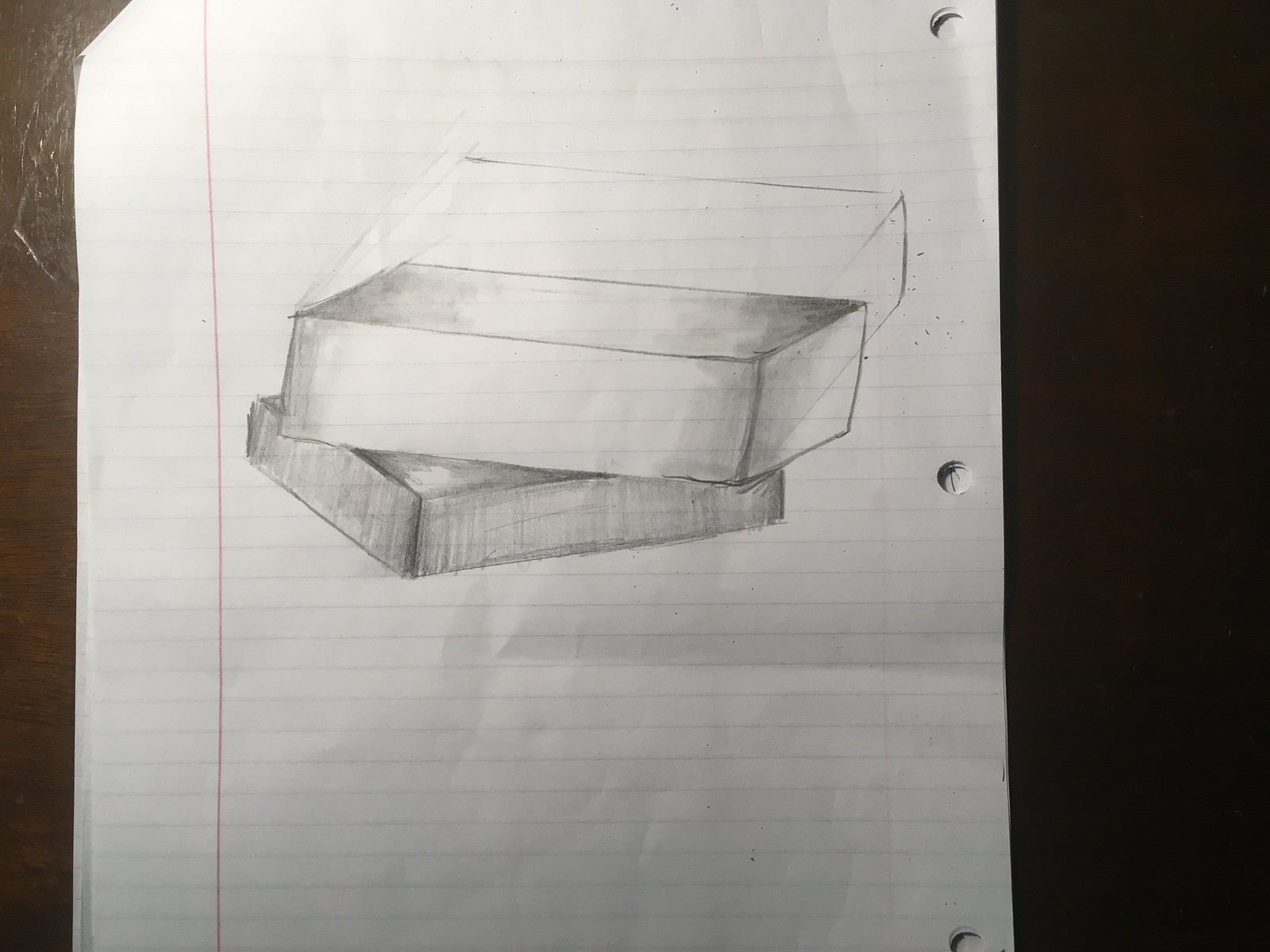This photograph captures a pencil sketch done on several sheets of lined loose-leaf paper, which are slightly misaligned and three-hole punched on the right side. The drawing depicts two brick-shaped blocks positioned on top of each other, with significant shading to provide depth and texture. The top block, thicker and more unevenly placed, appears partially erased, revealing some pencil smudges. The lined pages also feature a folded-over top left corner, and rest on a shiny, dark brown surface. The sketch, executed in black and gray pencil, employs a three-dimensional style to give the simple blocks a somewhat realistic appearance.